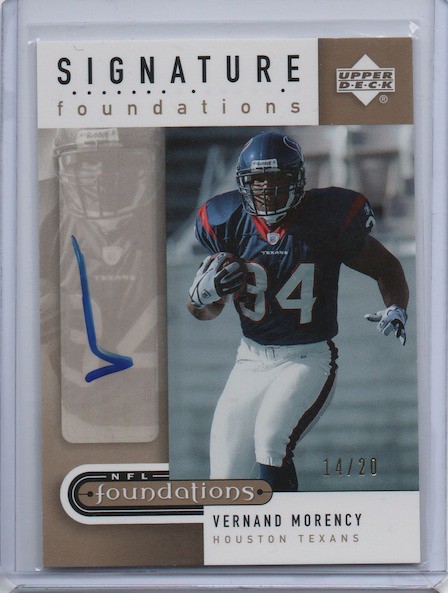This photograph showcases a signed football trading card encased in a clear plastic protector, resting on top of a white book. The card is branded by Upper Deck and labeled "Signature Foundations." At the top of the card, "Signature" is written in black text, with "Foundations" in brown or gray text below it. To the top right, the Upper Deck logo is prominently displayed. The color photograph on the card features an African American male athlete, Vernand Morency, wearing a blue and red football uniform with the number 34 in white, along with a blue helmet, white pants with black stripes, and white and black gloves, as he runs on a football field holding a brown football. The player's team, "Houston Texans," is indicated in brown text beneath his name, which is printed in black text on a white background. The card also has "14/20" marked in gold in the lower section, signifying its limited edition status. The overall image includes additional elements like a bookmark and a check on the left side.